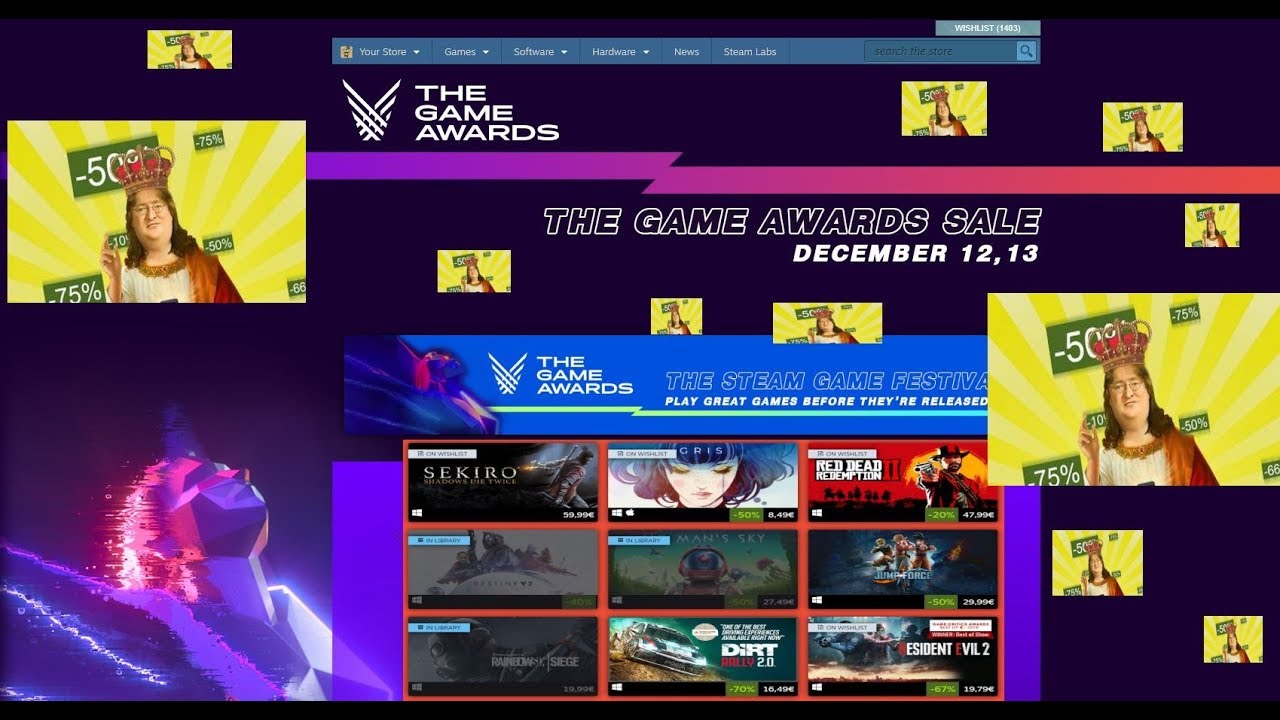Screenshot of a dark-themed website showcasing the Game Awards sale with a predominantly black background interspersed with hints of blue. The highlighted image features an individual with long hair and glasses, crowned with a red velvet crown, possibly depicted in cosplay attire. This image is repeated multiple times across the site, appearing on the left side, top right corner, the center, and right side in various sizes. Superimposed on these images are discount percentages “50%” and “75% off,” highlighting the ongoing sale from December 12th to 13th.

At the bottom, a blue text box announces the Steam Game Festival, emphasizing the opportunity to "Play great games before they're released," accompanied by several game thumbnails. Above this, a teal-colored navigation menu is centered at the top of the page, listing options like 'Your Store,' 'Games,' 'Software,' 'Hardware,' 'News,' and 'Steam Lab.'